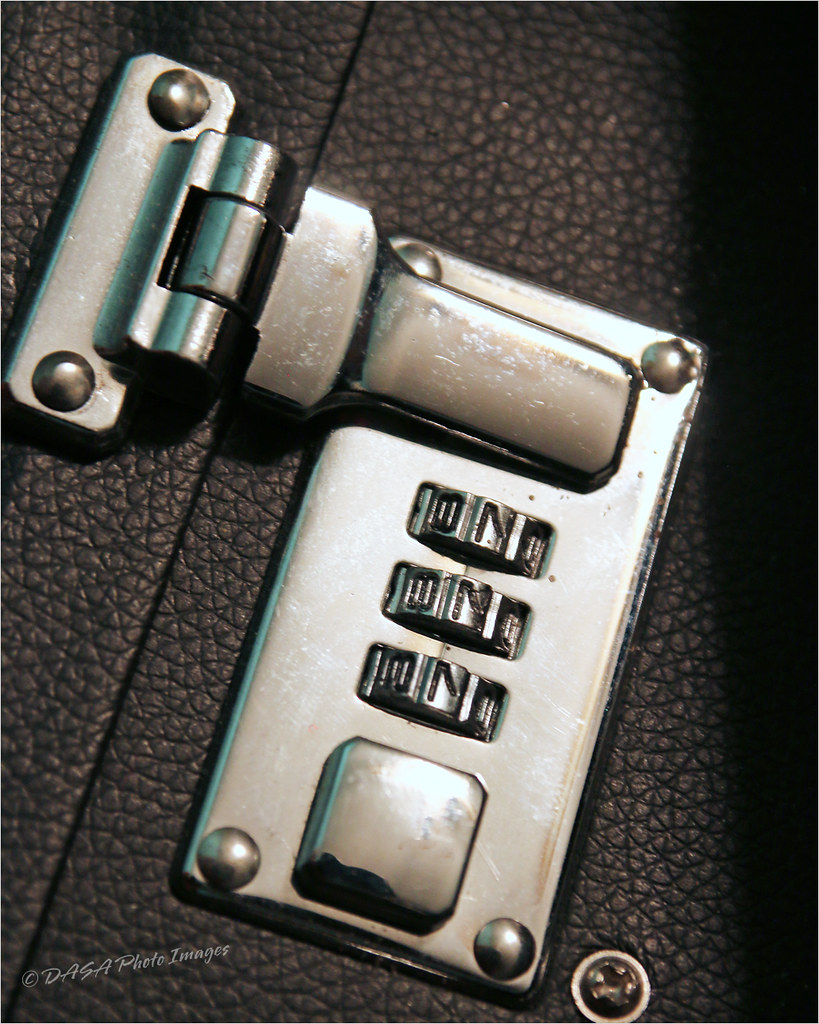This image is a detailed, close-up photograph of a combination lock on a black leather briefcase. The material of the briefcase is either real or imitation leather with a textured finish. The lock mechanism is positioned prominently in the center of the image. On the left side, there's a sturdy, steel-colored hinge with rivets securing it to the briefcase. This hinge features a long tongue that fits into the rectangular slot on the right side, where the combination lock is situated.

The combination lock itself is a vertical design with three dials. Interestingly, these dials are set to the combination 777, which stands out numerically. Once the correct combination is set, a square release button next to the dials can be pressed to unlock the clasp. The mechanism also includes a Phillips head screw in the bottom right corner, providing additional security to the lock assembly.

Furthermore, the image includes a watermark at the bottom left corner, which reads "DASA photo images" in a small, white italic font. This watermark adds a touch of authenticity and professionalism to the photograph. Overall, this close-up shot meticulously captures the intricate details of the briefcase and its locking mechanism.